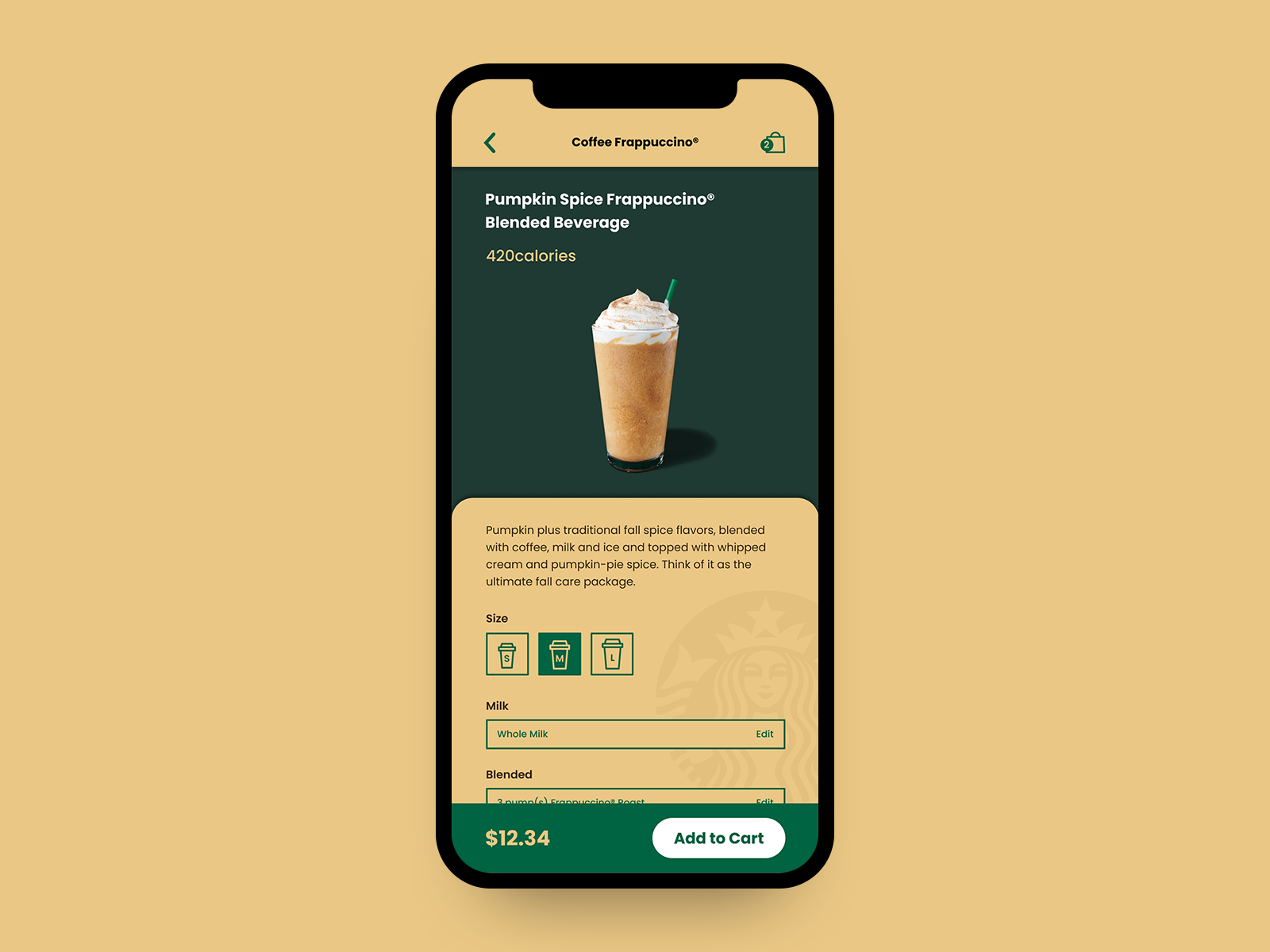Centered in this image is a mobile device showcasing a detailed description of a beverage, set against a vibrant orange background. Dominating the screen is an enticing depiction of a pumpkin spice frappuccino, emphasized by the text around it. 

Visible in the middle of the image is a coffee cup filled with a creamy pumpkin spice frappuccino, topped generously with whipped cream and a sprinkle of pumpkin pie spice. The beverage is described as a blend of pumpkin and traditional fall spice flavors, mixed with coffee, milk, and ice. 

Additional text highlights the drink's details: size medium, made with whole milk, and containing 420 calories. The price of this autumnal delight is noted as $12.34. The device interface features vibrant accent colors, including orange, green, and white, enhancing the fall-themed presentation of this blended beverage, advertised as the ultimate fall care package.